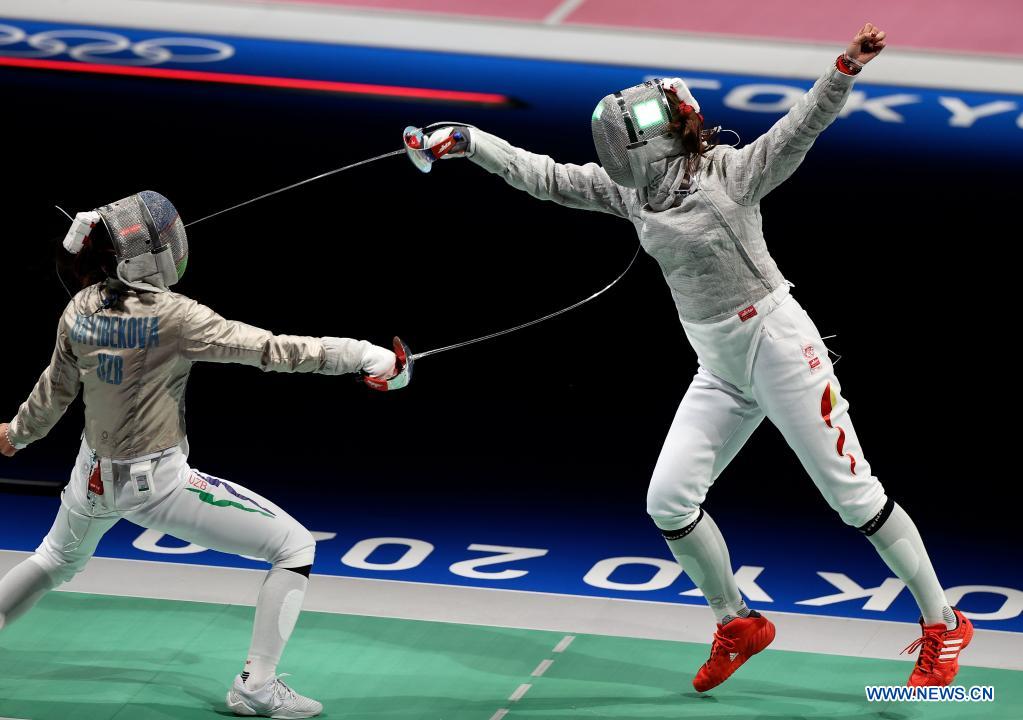In this indoor image, two people are engrossed in a fencing match on a light green mat with white lines, set against a blue and pink background. The background prominently features the Olympic emblem, indicating this could be a competition at the Tokyo Olympics, with partially visible text reading "Tokyo 2020." Both athletes are equipped with traditional fencing gear: their gray masks have a mesh design protecting their heads and faces, while their gray vests and white pants ensure optimal mobility and safety. One fencer sports red shoes, the other has white, low-fitting tennis shoes. The fencer on the right wields a silver-colored sword with a red handle in their right hand. The pants of the right fencer also exhibit logos and artwork. At the bottom right of the image, the website "www.news.cn" is visible in blue font with a white border. The setting's dynamic interplay of colors and details lends an intense atmosphere to this high-stakes duel.